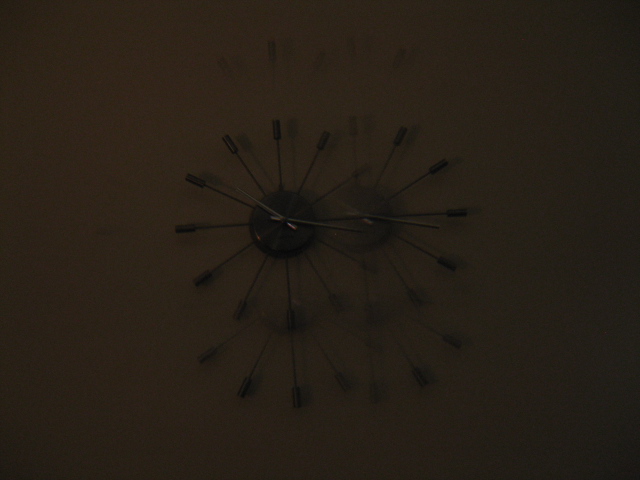The image depicts a dimly lit, chocolate brown and dark gray interior of a house with a decorative clock mounted on a yellowish wall. The clock itself has a minimalist, starburst design with gold hands pointing in different directions and lacks traditional numbers, instead featuring individual strands with thicker tips at each point. There seem to be reflections or shadows suggesting the presence of additional clocks or overlapping shadows, especially noticeable to the right, giving the appearance of multiple, slightly faded clocks. The central part of the clock is a small, round black circle, contributing to the abstract and surreal quality of the image.